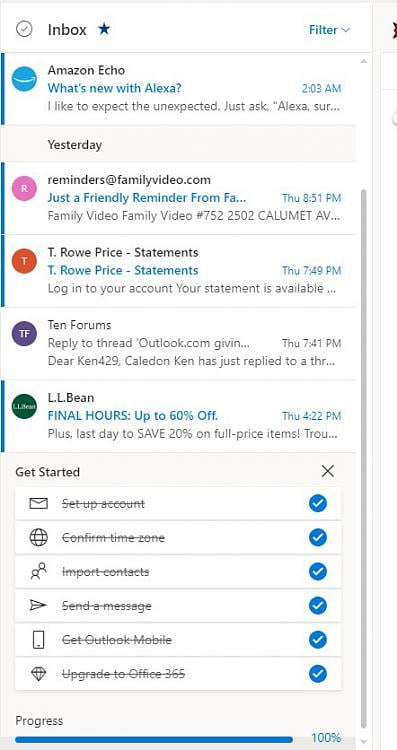The depicted image shows a detailed view of an email inbox, specifically Gmail. At the very top, the header clearly states "Inbox," and there's an adjacent dropdown menu labeled "Filter." The first email in the inbox queue is from Amazon, titled "Amazon Echo: What's new with Alexa?" and was received at 2:03 a.m. The second email, received yesterday, is from familyvideo.com with the subject line, "Just a friendly reminder from FA..." Following that is an email from T. Rowe Price labeled "Statements." Further down, there's an email from forums@outlook.com with a truncated subject line, "Reply to thread..." The next email from L.L. Bean announces "Final hours: Up to 60% off." Below these, there's a section titled "Get Started" featuring a checklist that indicates this is Outlook's setup process. Every item on the checklist is marked complete, including "Set up account," "Confirm time zone," "Import contacts," "Send a message," "Get Outlook mobile," and "Upgrade to Office 365."